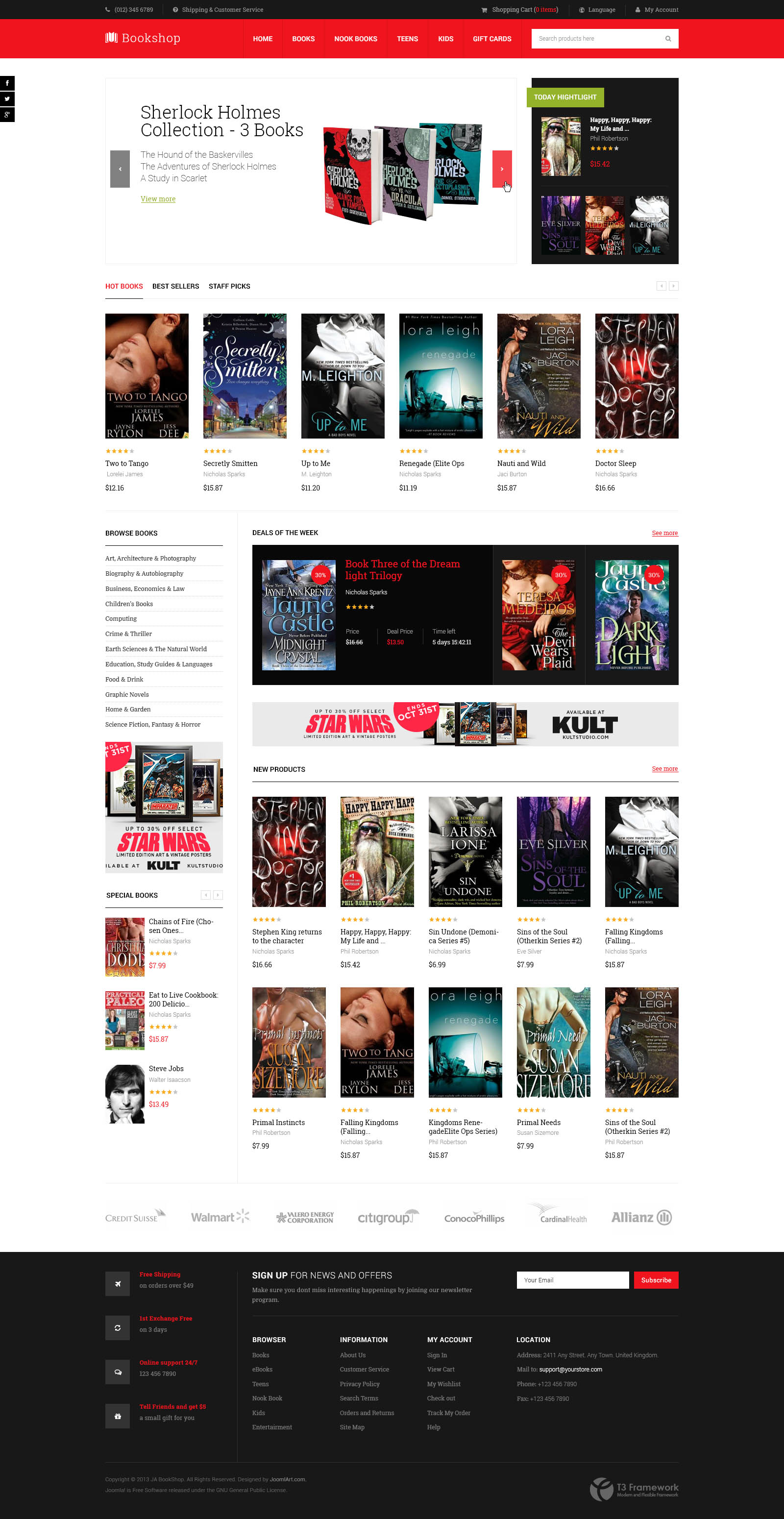The image depicts the homepage of a website named "Bookshop." At the top, a prominent red banner features the website's name alongside clickable options labeled Home, Books, Nook Books, Teens, Kids, and Gift Cards. Below this banner, there's a white search bar for product searches. Additionally, icons and links for a shopping cart, language settings, My Account, Shipping, Customer Service, and a contact phone number are displayed in black across the top.

The main content area highlights the Sherlock Holmes collection, featuring three classic titles: "The Hound of the Baskervilles," "The Adventures of Sherlock Holmes," and "A Study in Scarlet." These books are prominently displayed with their covers.

A "Today Highlight" section below showcases a variety of books, categorized into Hot Books, Best Sellers, and Staff Picks. Currently, the Hot Books category is selected, displaying book covers, prices, and authors' names.

Further down, there's a section labeled "Deals of the Week," presenting current book deals, and another section for New Products, which includes book ratings, titles, authors’ names, and prices.

On the left-hand side, there’s a feature for Special Books. At the very bottom of the page, a black box offers additional navigation options.